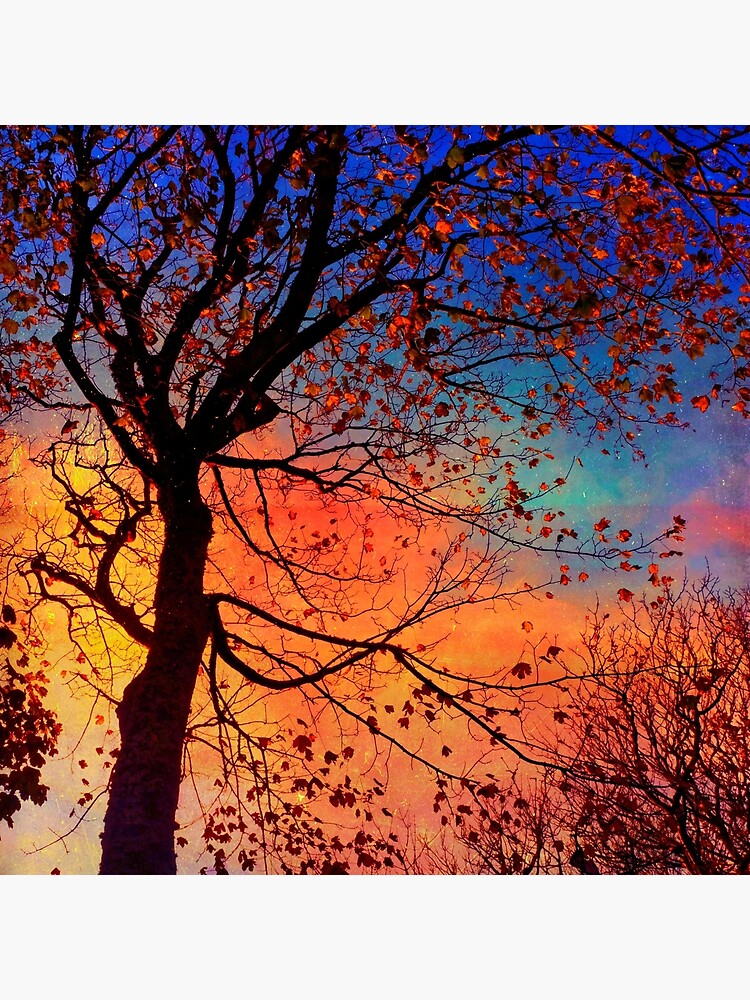This vibrant image, which could be either a photograph or a highly realistic painting, captures the transitional beauty of either sunrise or sunset. The sky showcases a stunning gradient, with a deep blue at the top fading into a greenish-blue tint, and then blending into rich oranges and yellows towards the lower left. Dominating the scene is a tall, black tree with a thick trunk positioned on the left side; its intricate network of branches extends all the way to the smaller shrub on the right, which is also characterized by dark, barren branches. The foliage on the main tree and shrub highlights the essence of fall with sparse, brilliant red, brown, and orange leaves, contrasting against the dark, thin branches and the sky's vibrant hues.